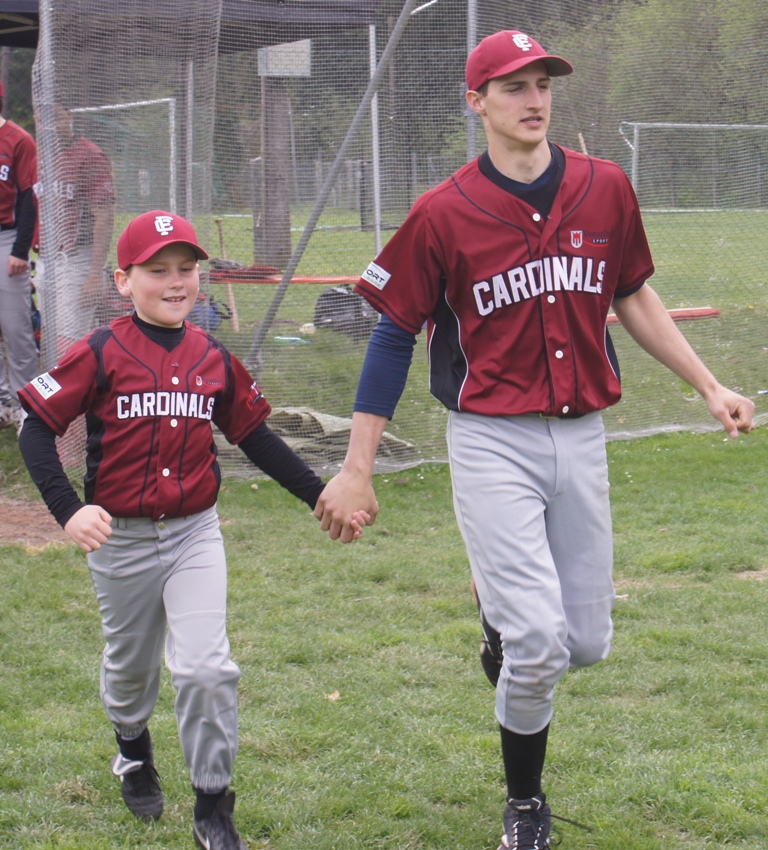The image captures a heartwarming scene of two boys holding hands as they walk towards the viewer. Both are dressed in matching baseball uniforms, including red jerseys with "Cardinals" written in white letters, red baseball hats, and white baseball pants. The shorter boy on the left, approximately 10 years old, wears a black long-sleeve shirt under his jersey, while the taller boy on the right, who looks to be around 16, sports a blue long-sleeve shirt. Each wears black sneakers. They walk on green grass, with a white mesh fence and additional players in similar uniforms as a backdrop. To the left, there is an orange bench, a wooden baseball bat, and several bags likely containing more baseball gear. The scene is set on a baseball field, capturing a moment of camaraderie and togetherness.